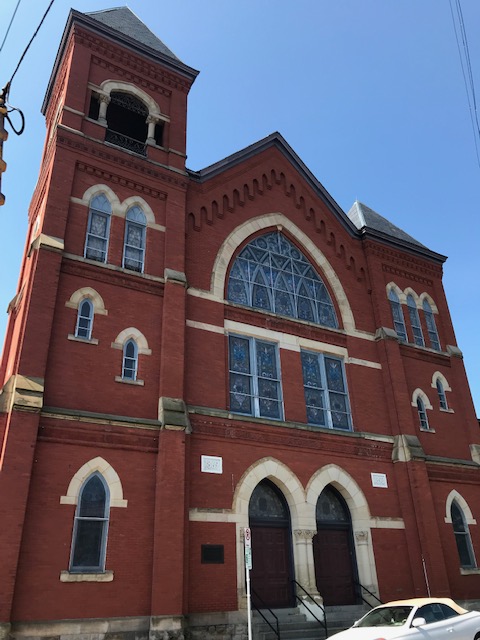The photograph captures a charming red-bricked building that strongly resembles an English-style church. The focal point of the structure is its array of stained glass windows, notable for their pointed, arched tops and framed in white stone or marble accents. The building features two distinct towers flanking the main structure; the left tower rises an additional floor, possibly functioning as a bell tower, complete with an opening resembling a balcony, while the right tower is capped with a pointy roof. The architectural design, though not overly intricate, exudes a certain grandeur and historical charm. Steps lead up to the double-arched doorways at the front, all set against a backdrop of a clear blue sky. Parked directly in front of the church is a white sedan, enhancing the serene, well-maintained appearance of the scene.